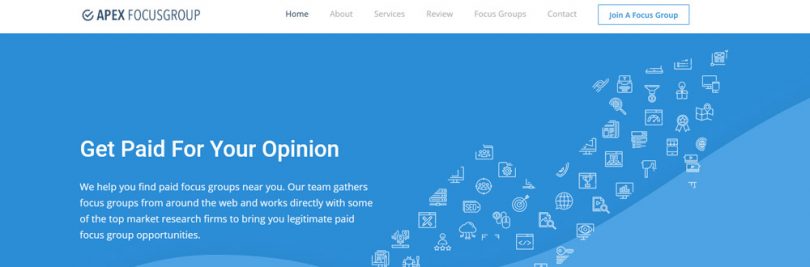Here is a detailed and cleaned-up description for the given image:

---

The screenshot captures a section of a web page featuring a dark blue and lighter blue wave gradient as its background. In the top left-hand corner, there's a bold title "Apex," accompanied by a check mark encircled for emphasis. Adjacent to it, "Focus Group" is displayed in gray text.

The navigation menu below is organized in bold and regular text:

- **Home** (bold)
- About
- Services
- Review 
- Focus Groups
- Contact

A blue box highlighted with bold text reads "Join a Focus Group."

Central to the image is a prominent banner with the text "Get Paid for Your Opinion" in bold white lettering, followed by a smaller white font explaining, "We help you find paid focus groups near you. Our team gathers focus groups from around the world and works directly with some of the top market research firms to bring you legitimate paid focus group opportunities."

Alongside the textual content, there's a creatively designed arrow composed of various small icons. This arrow has a dynamic path—upward, then downward, and upward again—and features an arrowhead. The icons forming the arrow include representations related to the World Wide Web, Google Rewards, reminders, graphs, appliances, and electronic devices like a computer monitor and a cell phone.